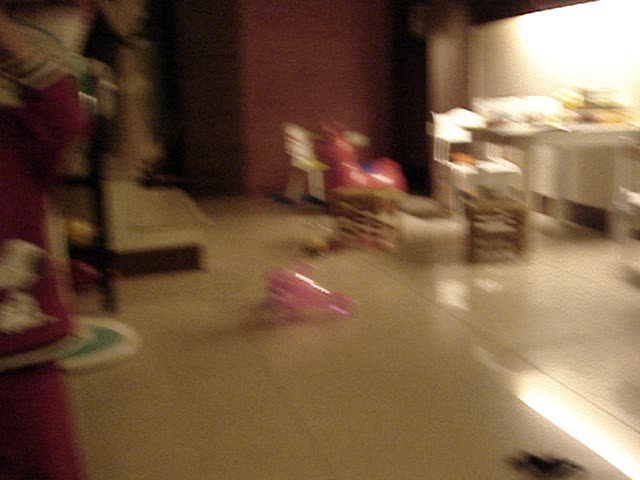This highly blurred photograph appears to capture an interior space that might be a playroom or a section of an office building repurposed for children's activities. The floor, an off-white or yellowish hue, has a shiny finish, contributing to the room's illuminated and spacious feel. On the right side, there's a white cabinet standing against a predominantly red back wall, providing contrast to the room's overall color scheme. Amidst the blur, a pink object and what looks like a rocking horse are discernible, suggesting this area is designed for play. To the left, an indistinct structure that could be a shelf is visible, though its contents remain unclear due to the photograph's low resolution. Overall, the scene hints at a playful yet organized environment meant for children.